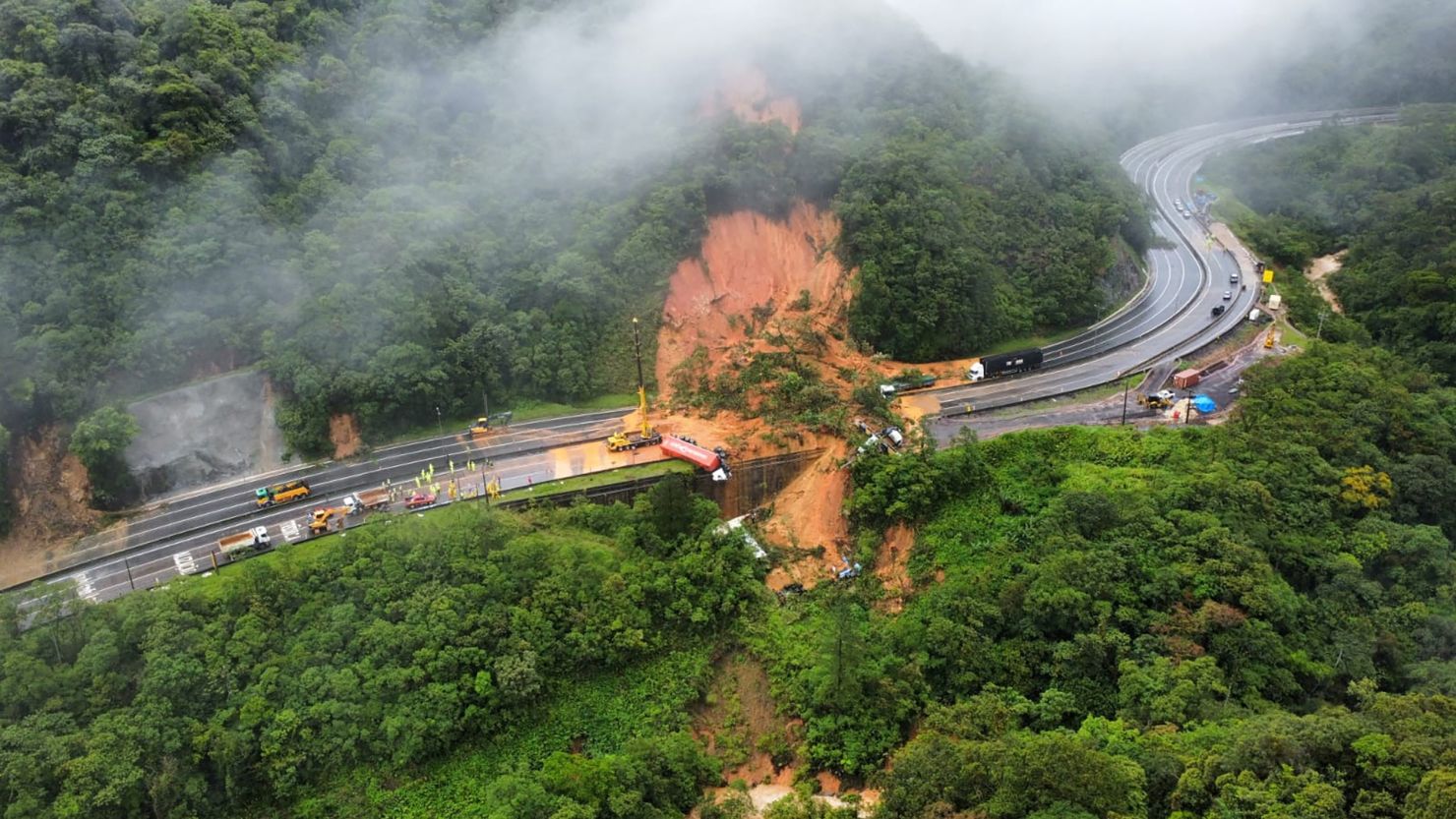This is a detailed aerial photograph of a hazardous landslide on a curving, multi-lane highway weaving through a lush, mountainous forest. Dense green foliage covers the surrounding area, with patches of trees and bushes, creating a humid and foggy atmosphere. The landslide has unleashed a cascade of orangish-tan dirt and debris across the roadway, blocking a significant portion of it and causing several vehicles to be pushed off the edge. Notably, a red truck is lying on its side precariously near the cliff’s edge, while other vehicles are halted behind it. Emergency response crews and their trucks, including a giant crane, are actively working to clear the landslide and manage the situation, with some smoke visible from their activities. The scene is one of natural upheaval and focused human effort amidst a sprawling green landscape disrupted by the dramatic landslide.